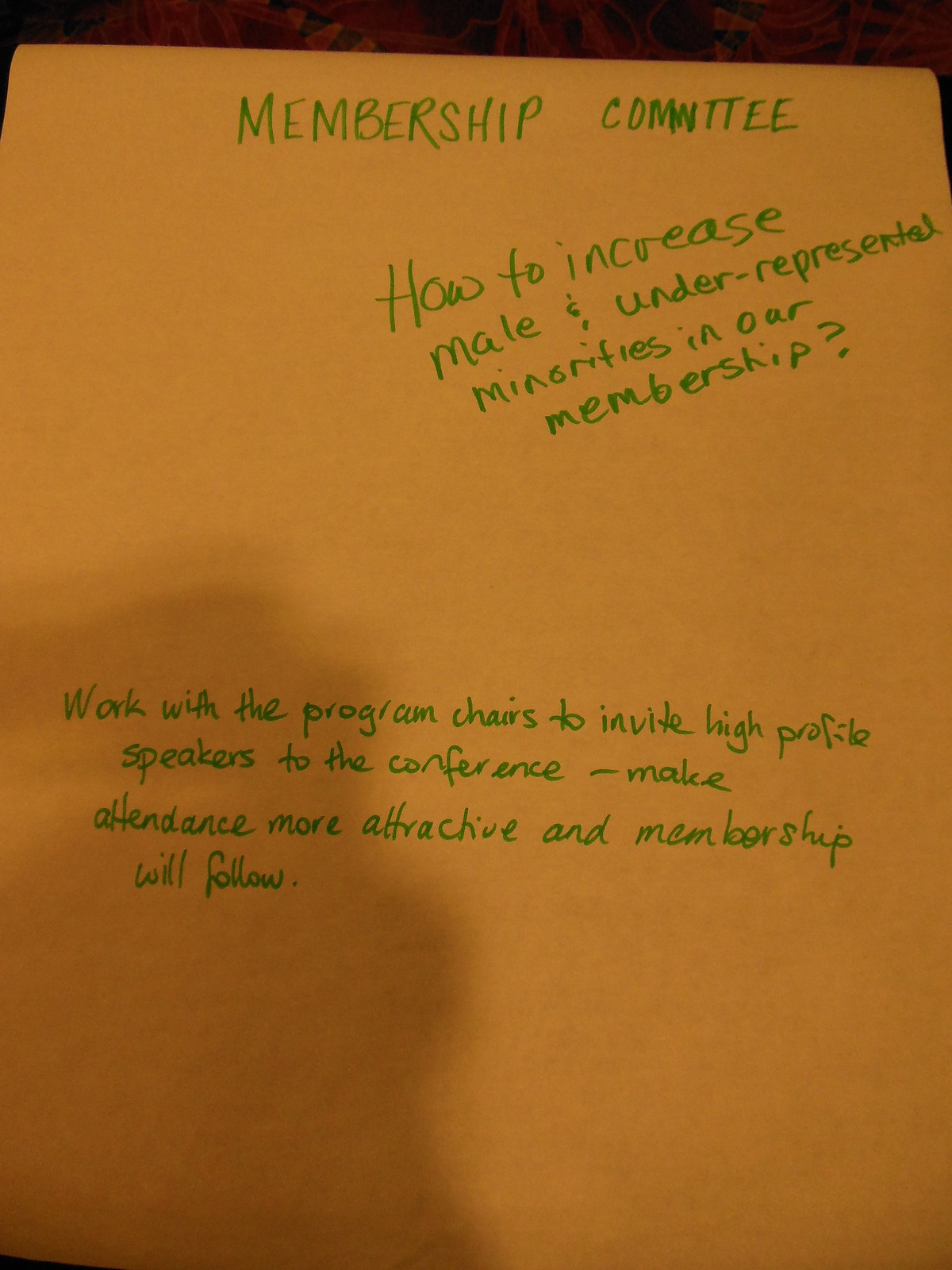The photograph captures a large sheet of yellow paper typically used on an easel for team-building sessions or brainstorming activities. The background features a patterned wooden desk, although the dim lighting and a shadow—likely from the person's hand or phone—make the pattern hard to discern. At the top of the paper, "MEMBERSHIP COMMITTEE" is boldly written in uppercase letters with a green marker. Centered below and angled slightly to the right, it reads: "How to increase male and underrepresented minorities in our membership?" Following that, roughly a paragraph lower and centered, is a statement, also in green marker: "Work with the program chairs to invite high-profile speakers to the conference - make attendance more attractive and membership will follow."